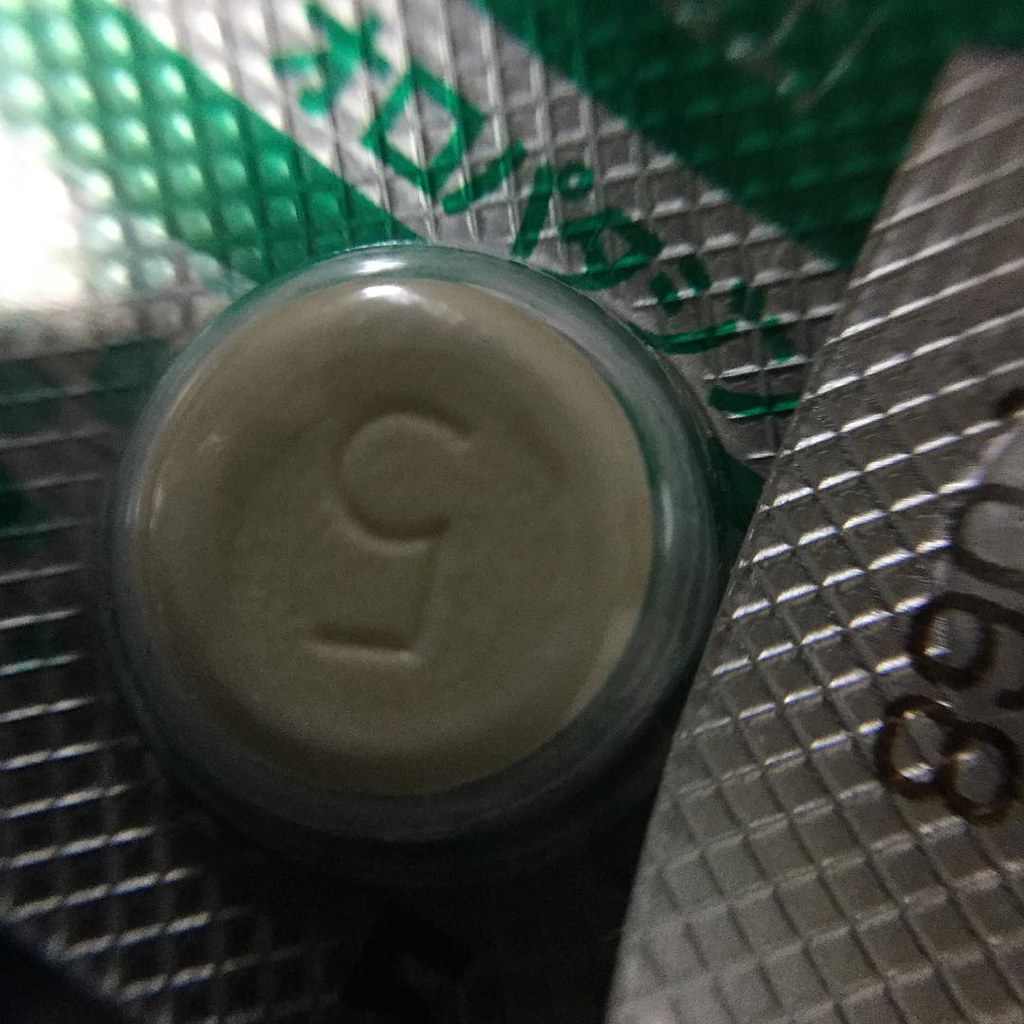This extreme close-up photograph features two overlapping blister packs. The top blister pack has a silver grid pattern with black-printed numbers, prominently displaying "eight," "nine," and "zero" towards the right edge, as well as "six" further in. The underlying blister pack showcases a silver surface with bright green stripes and text in a foreign language, also in bright green. Both packs have a ridged and shiny foil texture. Dominating the left side of the image is a plastic blister bubble containing a circular, cream-colored pill with the number "five" engraved upside down in its center. The intricate details and textures of the blister packs and pill are accentuated by light reflections, adding depth to the overall metallic and rigid appearance.